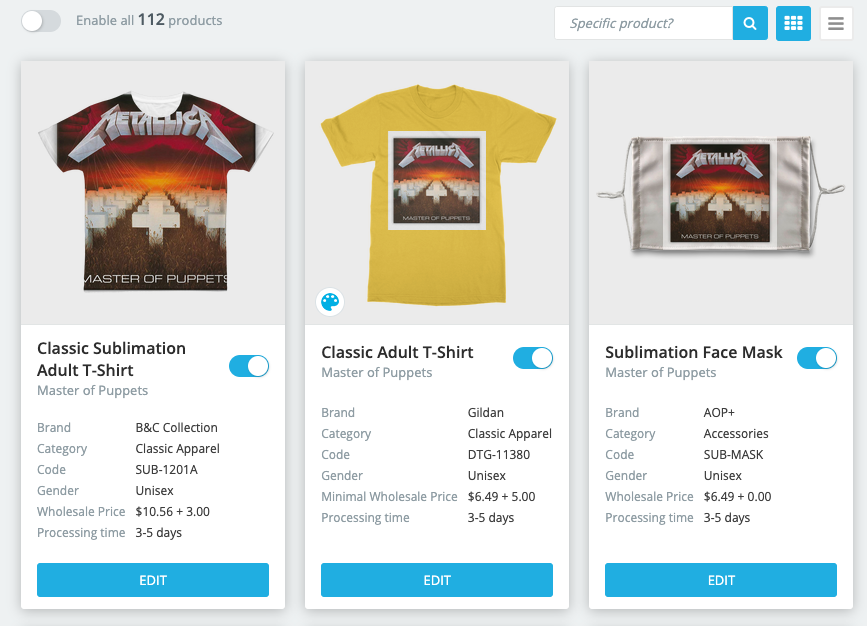This screenshot shows a section of an apparel website featuring three Metallica-related items from the "Master of Puppets" collection. 

On the left, there is a toolbar displaying 112 products available, a search bar, and options to customize the view of the results. The main focus of the screenshot is on three vertical panels with drop shadows, each showcasing a different piece of merchandise.

1. **Classic Sublimation T-Shirt**:
    - Design: Full front, collar, and sleeves adorned with the "Master of Puppets" album cover.
    - Brand: BNC Collective
    - Category: Classic Apparel
    - Code: SUB-1201A
    - Gender: Unisex
    - Wholesale Price: $10.56 plus $3 processing
    - Processing Time: 3 to 5 days
    - Additional Feature: Blue "Edit" button underneath.

2. **Classic Adult T-Shirt**:
    - Design: Smaller "Master of Puppets" album cover with a white border, presented on a yellow t-shirt.
    - Brand: Gildan
    - Category: Classic Apparel
    - Code: DTG1130
    - Gender: Unisex
    - Wholesale Price: $6.49 plus $5 processing
    - Processing Time: 3 to 5 days

3. **Sublimation Face Mask**:
    - Design: "Master of Puppets" album cover printed on the mask.
    - Brand: Accessories
    - Category: Sublimation Face Mask
    - Code: Sub-Mask
    - Gender: Unisex
    - Wholesale Price: $6.49, no additional processing cost
    - Processing Time: 3 to 5 days
    - Additional Feature: Blue "Edit" button underneath.

Each panel is meticulously detailed, providing all necessary product information including pricing, processing times, and product codes, effectively catering to potential bulk buyers or retailers.